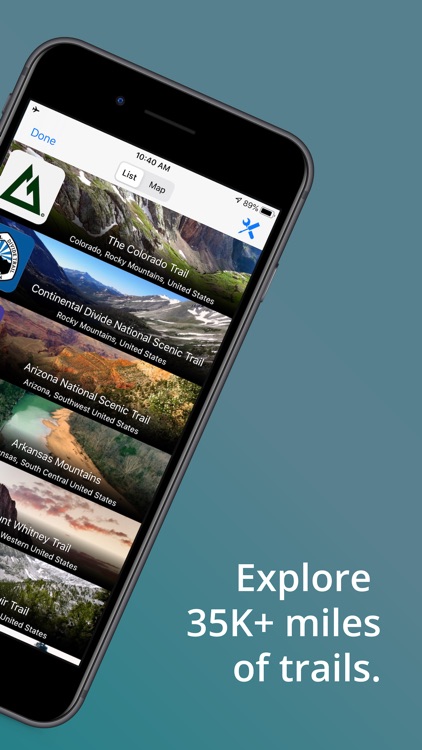A screenshot of a promotional advertisement features a minimalist design with a gray rectangle as the background. A smartphone is partially visible, emerging from the left side of the frame at a slight rightward tilt. The bottom-left corner of the phone is cut off, leaving about three-quarters of the device in view. 

The text within the gray rectangle reads, "Explore 35,000 miles of trails," displayed prominently in white letters.

On the smartphone's screen, the top bar indicates the time is 10:40 AM, and the battery level is at 89%. Below this, there is a list of trails, including:
- **The Colorado Trail**, accompanied by an image of moss-covered rocks.
- **The Continental Divide National Scenic Trail**, depicted with a photo of mountain peaks.
- **Arizona National Scenic Trail**, featuring vibrant fall-colored trees alongside evergreens in a mountainous landscape.
- **Arkansas Mountains** and **Mount Whitney Trail** are listed as well, while the text for another trail is obscured due to the cutoff corner of the phone.

This advertisement aims to entice viewers to explore various scenic trails using a dedicated app or service.